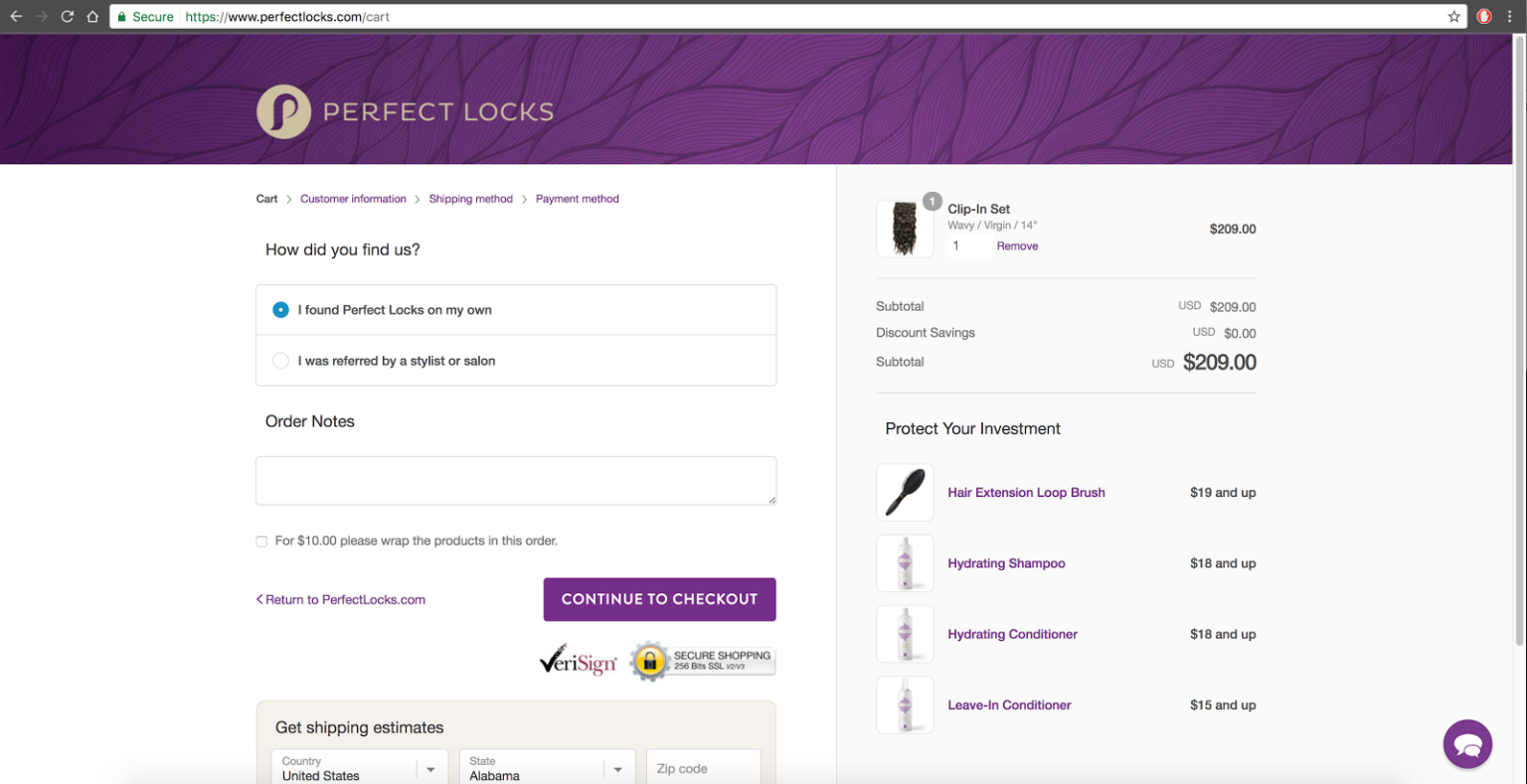A horizontally rectangular screenshot of the upper portion of a web page from the URL https://www.perfectblocks.com. The left side of the screen displays several sections starting with a prompt "How did you find us?" followed by selection options. Below this, there is a field for order notes, and a button labeled "Continue to Checkout" at the bottom. On the right side of the screen, the featured product is a "Clip-In Set" priced at $209. Directly beneath the product information, there's a promotional section titled "Protect Your Investment," which suggests four upselling items: a Hair Extension Loop Brush, Hydrating Shampoo, Hydrating Conditioner, and Leave-In Conditioner.